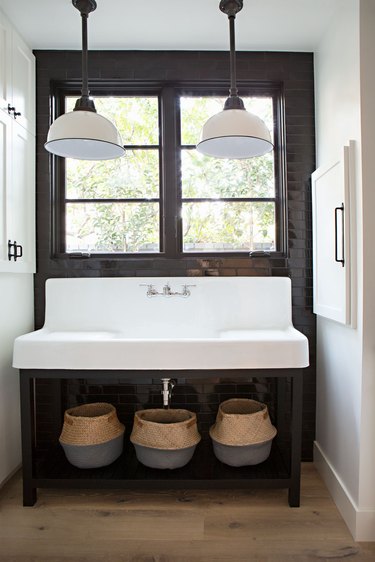This image depicts a modern farmhouse-style utility room with elements of both traditional and contemporary design. The room features white walls and a white ceiling, with a light brown hardwood floor that lends warmth to the space. The focal point of the room is an expansive, bright white porcelain sink that spans almost the entire width of the image. The sink has an elegant flat top curving down into the basin and is mounted on a black metal frame with a shelf underneath. This shelf holds three woven storage baskets, brown with matte grey undersides, providing both functionality and aesthetic appeal.

Above the sink, two large windows with black frames allow ample natural light to flood the room. The back wall, behind the windows and sink, is adorned with glossy black tile, contributing to the room's sleek and stylish look. Flanking the sink, on either side of the room, are white cabinets with simple black handles, offering additional storage space. 

Hanging above the sink are two pendant lights with white domed shades suspended from black rods, illuminating the area below. The combination of light wood flooring, black accents, and white elements creates a cohesive and inviting atmosphere, making this small utility room both practical and visually appealing.